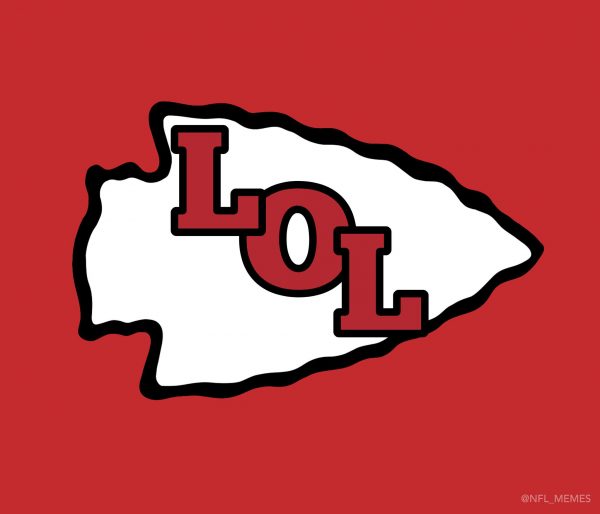The image appears to be a meme parody related to the Kansas City Chiefs. It features a square-shaped, dark red background. At the center of this background is a white arrowhead pointing to the right, bordered by a black, squiggly outline. Diagonally across the arrowhead, from the upper left to the lower right, are the letters "L-O-L" in large, dark red, capital letters, each outlined in black. At the lower right-hand corner of the red background, in small, translucent, white letters, is a watermark that reads "NFL_MEMES."